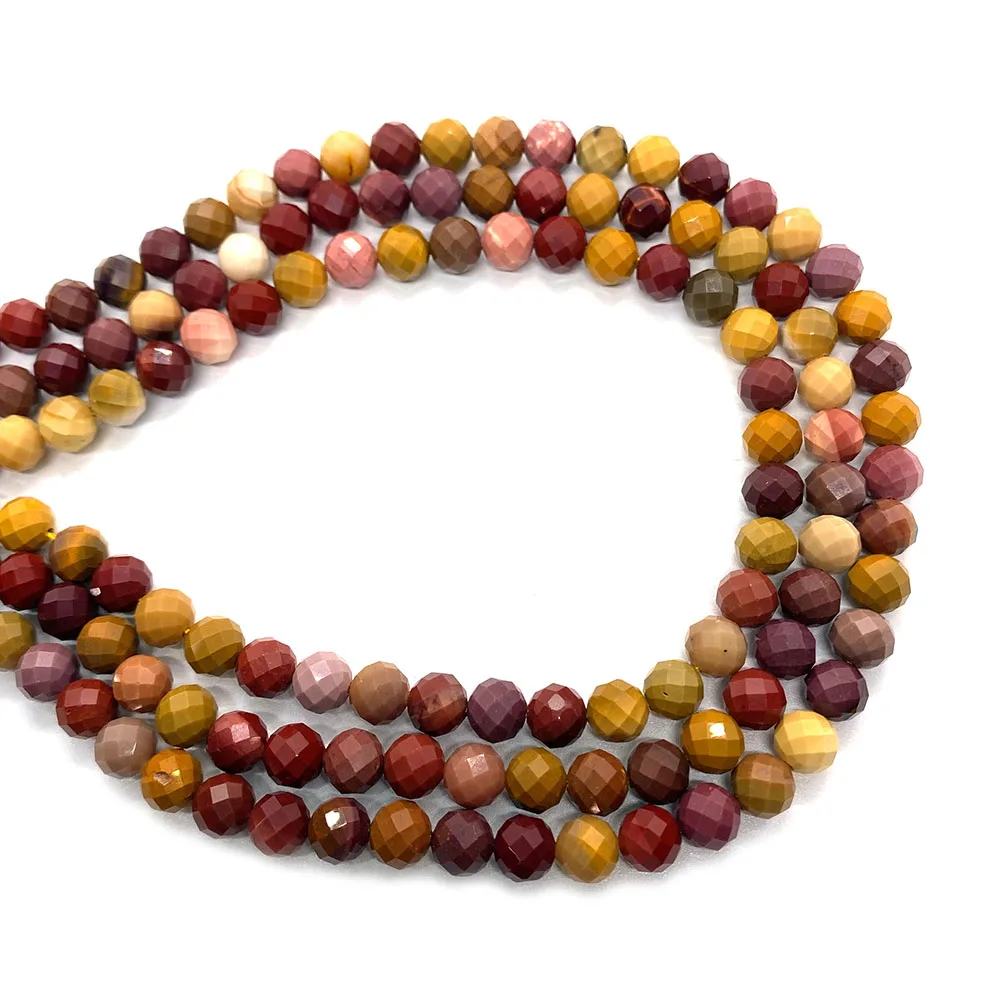The image features three intricately designed necklaces, arranged in a hood shape with their openings on the left side and their bottom parts on the right. These necklaces are placed in descending size—from the largest on the outside to the smallest on the inside. Each necklace is composed of ball-shaped beads, which have a multifaceted, honeycomb-like texture that catches and reflects light beautifully. The beads come in a diverse spectrum of colors, including yellow, light blue, dark blue, various shades of pink (from lighter to darker hues), and an assortment of browns (from lighter to darker shades). Additionally, there are hints of green, purple, off-white, cranberry, and white beads scattered throughout. The central areas between the necklaces reveal a white background. The image has a slightly digital and blurry quality, but the colorful, multi-surfaced beads are distinctly visible, adding to the overall vibrant and textured appearance of the necklaces.